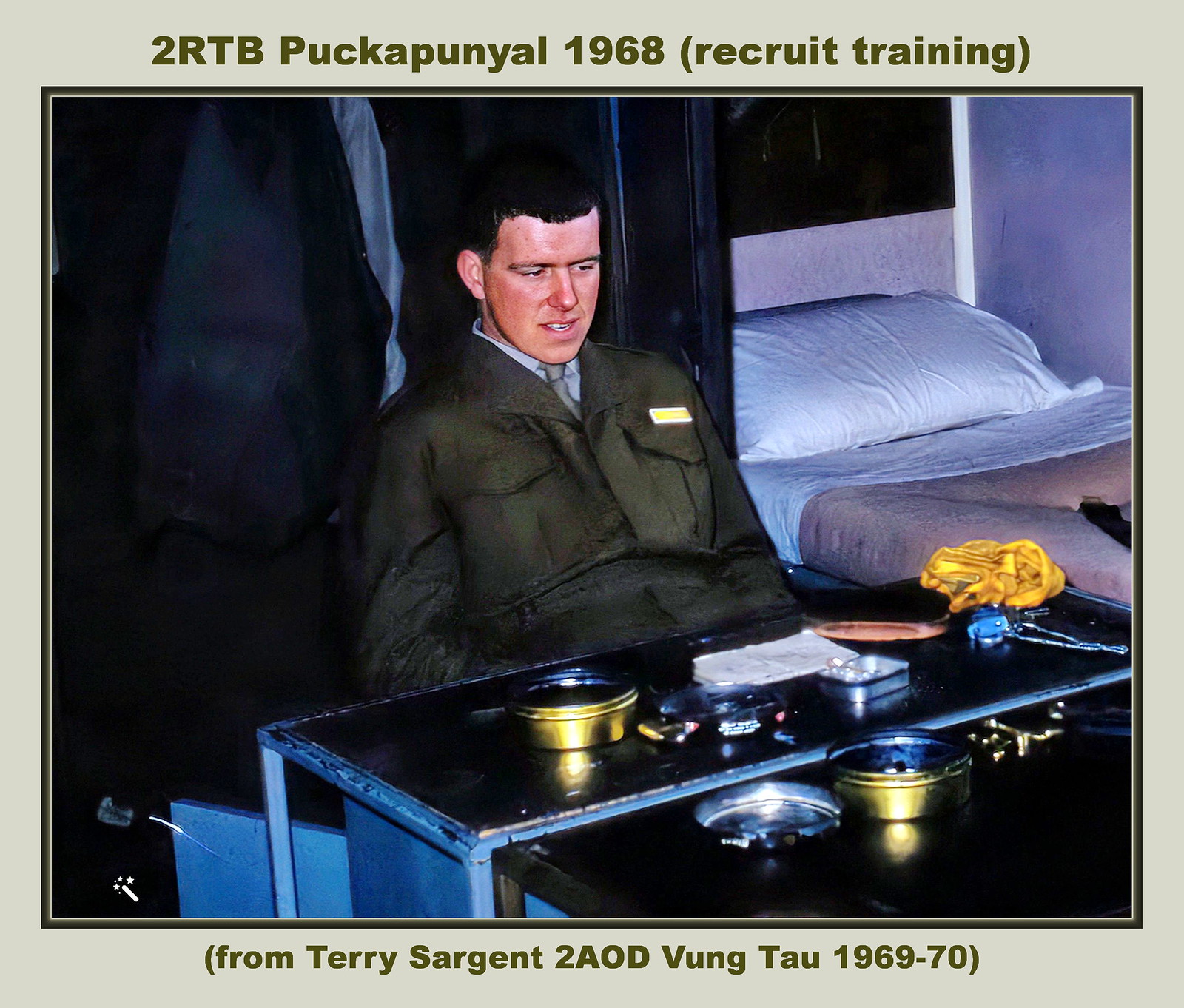The image is an old photograph from 1968-1970, depicting a military man inside a building. He has dark hair and light skin and is dressed in a green uniform with a yellow name tag, which is not readable due to the photo's quality. The man is seated at a desk cluttered with various items, including two golden containers with lids, a possible gold ashtray, and a yellow cloth or handkerchief. On the desk, there seems to be a lighter and some kind of chain among other indiscernible objects that he appears to be examining. To the right of the desk is a bed, made up with a pillow and a light pink blanket, indicating a typical military setup of the era. To the left of the man, there are coats or uniforms hanging. The photograph has text above and below the image: at the top, it reads "2RTB Puckapunyal 1968 (recruit training)" and at the bottom, in light green lettering, it states "From Terry Sergeant to 2AOD Vung Tau 1969-70."